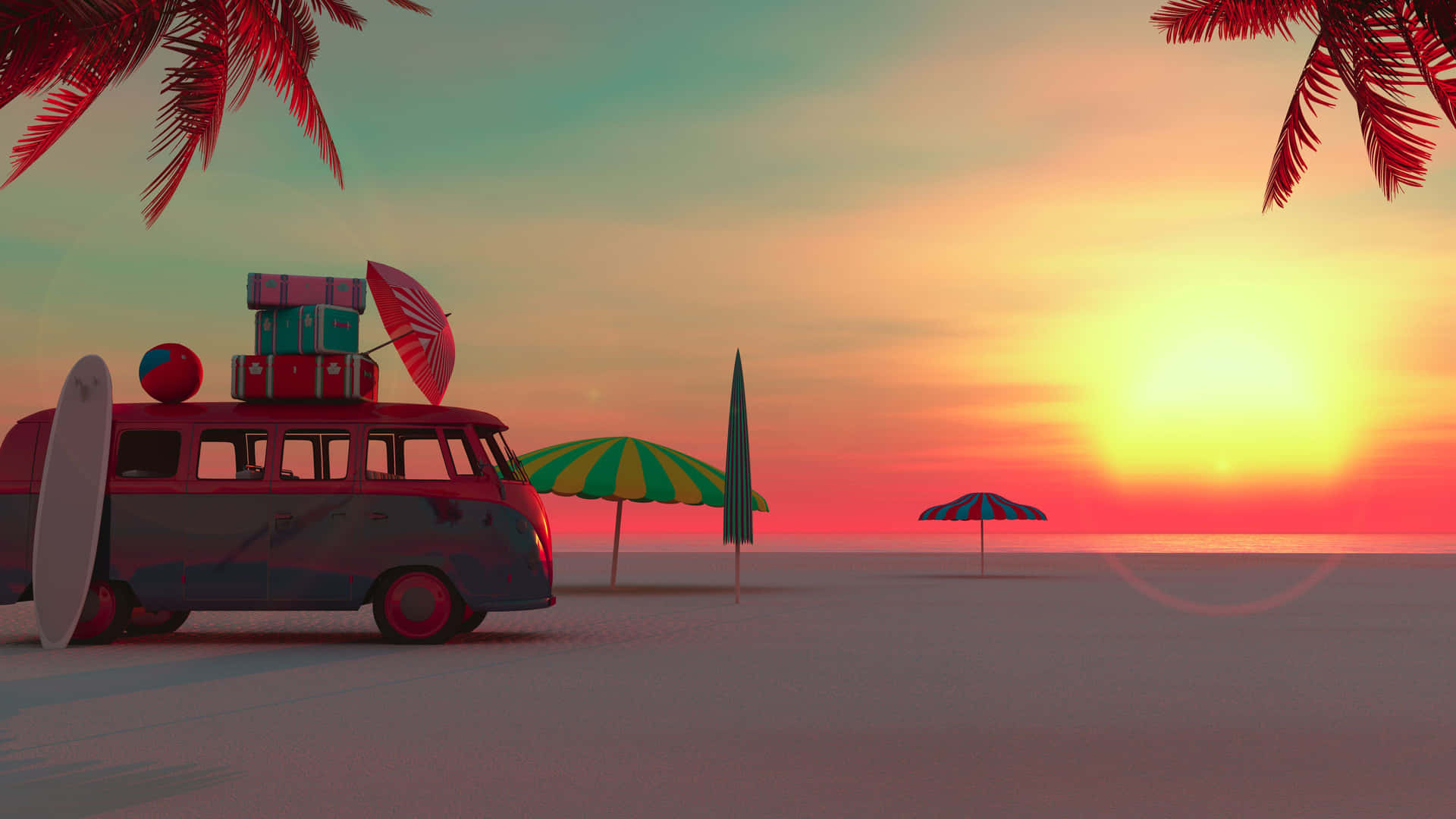This image portrays an AI-generated, high-contrast beach scene reminiscent of a cartoon or postcard. The colors are vividly bright and heavily saturated, adding to its artificial appearance. The flat, sandy ground of the beach is foregrounded by a setting sun visible on the horizon. The sky transitions dramatically from a pinkish hue near the horizon, through yellowy-orange, to blue at the top, creating a striking gradient. The ae sun is large and glowing yellow, casting a serene ambiance over the scene.

Nestled on the left of the image, a banged-up red and gray vintage BW van stands out. A tan surfboard leans against the van, while on its roof, three suitcases are precariously stacked — one pink, one teal, and one red. There's also a brightly colored beach ball in red and blue beside the suitcases. On the far left and right corners, palm trees frame the scene.

Scattered across the beach are several beach umbrellas: two open ones stick out from the sand and one closed, conical umbrella lying between them. Notably, a pink-and-white striped umbrella is set up near the van, highlighting the playful and relaxed beach atmosphere.